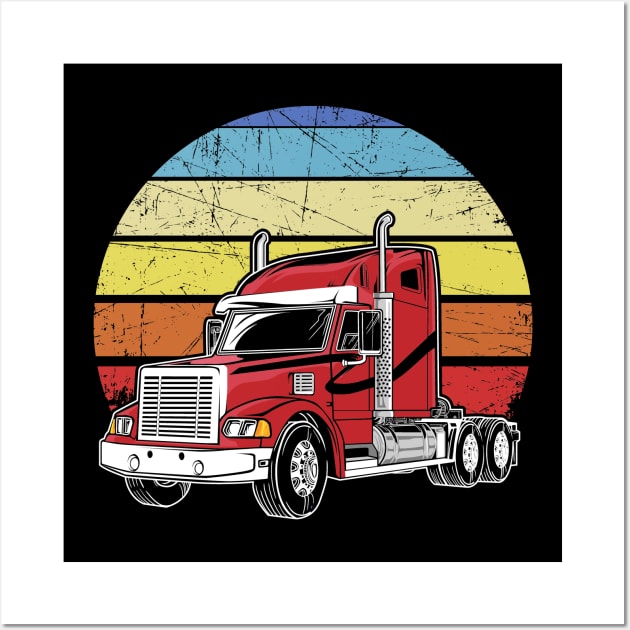This vibrant visual art piece features a black background framed by a white border. At the center of the composition is a horizontally striped, rainbow-colored circle in the following order from top to bottom: dark blue, light blue, tan yellow, bright yellow, orange, and red. Positioned in front of this colorful backdrop is a red semi-truck cab adorned with chrome detailing, including two smokestacks, a grill, and trim around the bottom. The cab has a distinctive black stripe running from the hood across the door. The truck is depicted at an angle, revealing two large black front tires and two smaller black back tires, all contributing to a striking pop-art aesthetic.